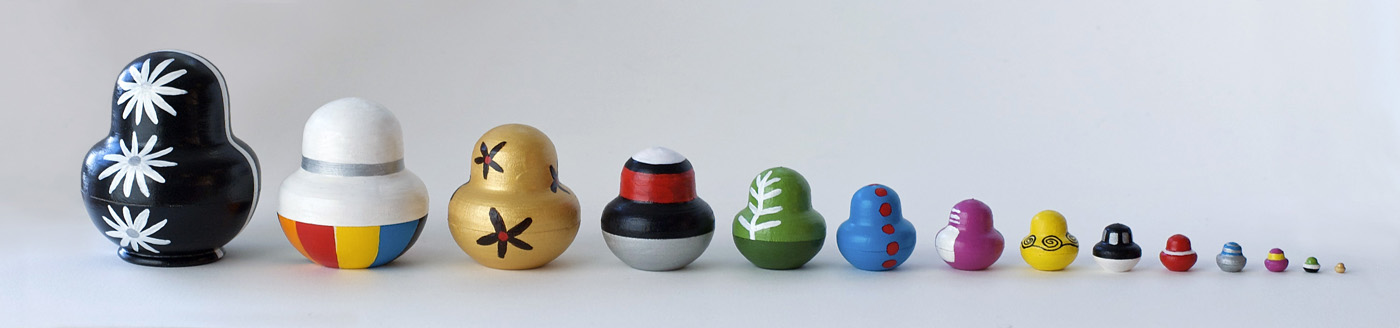The image features a set of matryoshka dolls arranged from largest to smallest, spanning horizontally across a gray background. These Russian-style nesting dolls, although faceless, boast a variety of intricate designs and vibrant colors. The largest doll on the far left is black adorned with three white flowers. Next is a white doll with a multicolored, beach ball-like base and a silver stripe running down its middle. Following that, a golden doll displays a couple of black stars. The fourth doll is decorated with alternating stripes of white, black, and red. Moving further right, the green doll in the middle sports a white plant design. A blue doll with red dotted lines comes next, followed by a pink doll featuring white accents. The eighth doll is yellow with a black spiral design. Subsequent dolls become increasingly smaller and include a black doll with a white base, a red doll with a white stripe, a silver doll with two blue stripes, a pink doll with a yellow band, another green doll with a white stripe, and finally, a small yellow doll. The entire array creates an eye-catching, gradient of colors and designs, all set against the uniform and neutral gray background.